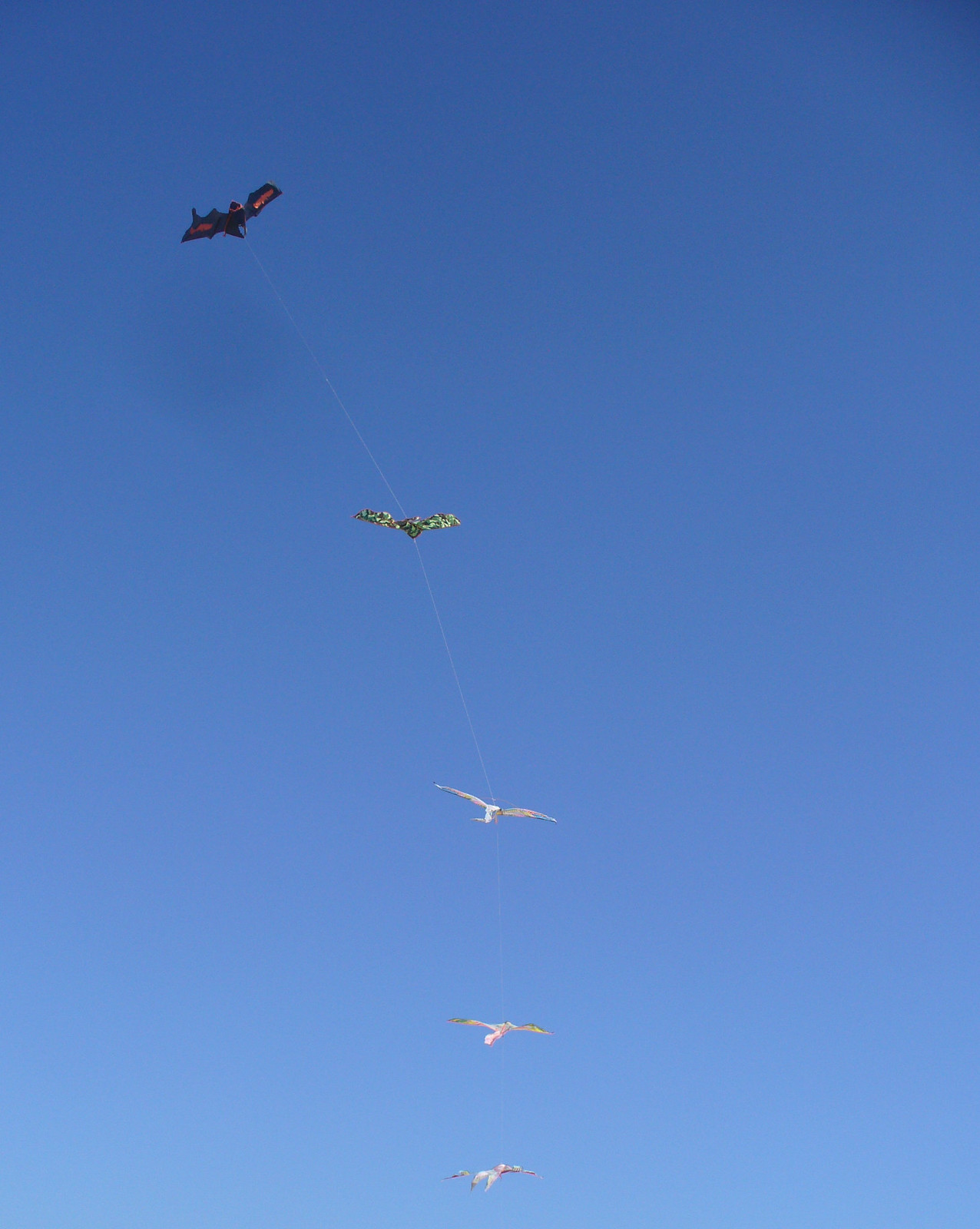The photograph features a vast expanse of clear, blue sky, unmarred by any visible infrastructure or boats. Dominating the scene is a string of five kites ascending high into the air, each attached to the same line. The kites are arranged sequentially, creating the illusion of a continuous train. Starting from the top, the lead kite is shaped like a bat, striking in its appearance with black and red markings around its eyes and wings. Following it are two more kites, each resembling white seagulls, spaced approximately 6 feet apart from each other. A fourth kite, slightly more distinct with green and brown hues, appears next in line. Concluding the sequence is another bat-shaped kite, this one predominantly black with red details. These kites present a mesmerizing aerial display against the pristine sky, capturing the essence of a serene yet whimsical moment.